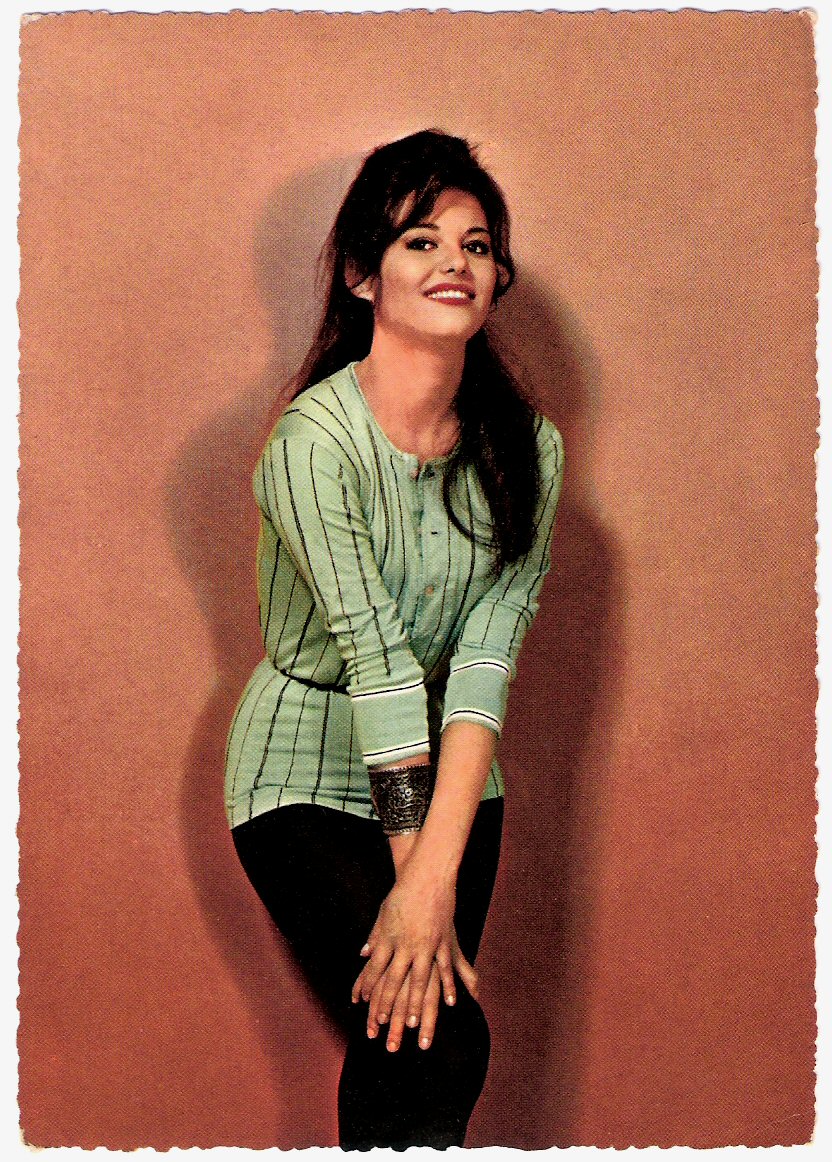The image is a highly stylized vertical photograph of a young woman against a light pinkish background, with her shadow visible. The woman, standing and slightly hunched over, poses flirtatiously with a smile. She has long brunette hair, styled in a half updo with some bangs, and it cascades about six inches below her shoulders, with her right side's hair behind her shoulder and her left side's hair in front. She wears striking red lipstick, accentuating her dark brown eyes. Her light mint green shirt, adorned with vertical black stripes, complements her figure. She is seen with a wide cuff bracelet just below her right elbow and is wearing black pants. Her pose is dynamic, with her right leg bent and both hands placed just above her right knee, overlapping. The color palette of the image primarily includes black, white, mint green, light pink, red, peach, and possibly a dark blackish brown.